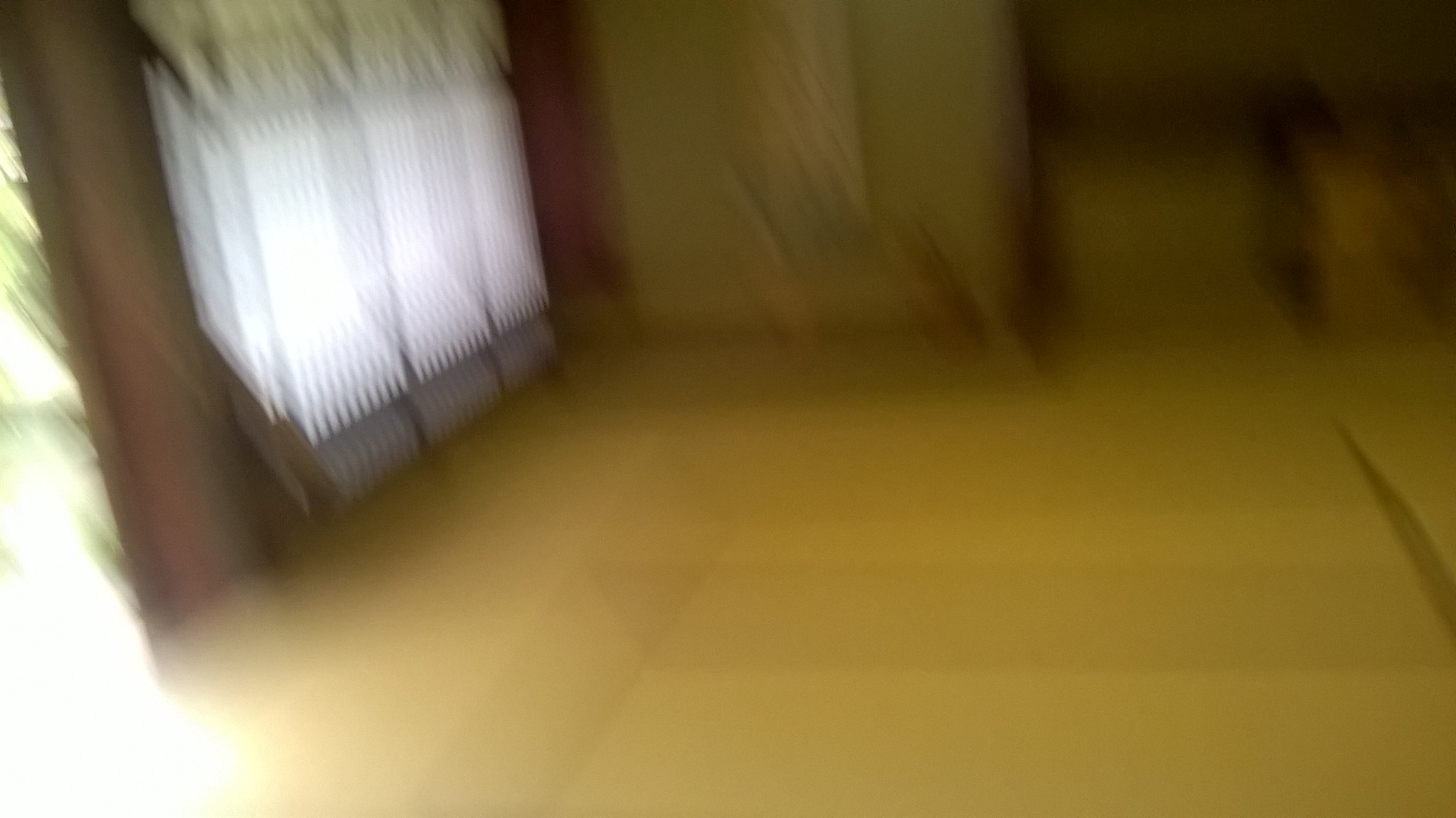The image depicts an extremely blurry room with indistinct boundaries and features, suggesting it was taken while the camera was in motion. The room appears to be largely empty, with the most discernible elements being a light source emanating from a doorway that possibly leads outside, and windows on the left-hand side with partially drawn blinds. The lower left corner shows a hint of green amidst the light, likely indicating the presence of trees or plants outside. The flooring is predominantly yellowish or beige, though any specific patterns or details are lost in the blur. In the upper right-hand corner, there are indistinguishable items that resemble boxes. The walls also take on a yellowish-beige hue. Overall, the brightest areas in the image come from the light filtering through the door and windows, while the rest of the room remains shrouded in shadow, further obscuring the finer details of the room's contents and layout.